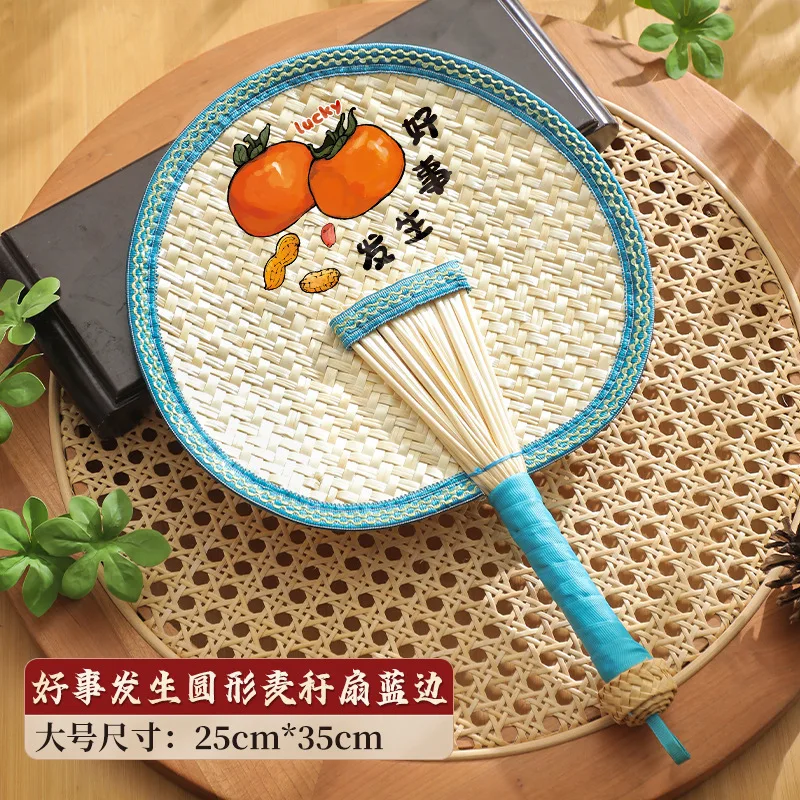This image showcases a woven, wicker-like paddle or fan with an off-white, cream-colored central area, adorned with detailed elements. Encircling the paddle is a light blue, almost teal border, which continues down into the handle. The handle transitions from a wider, V-shaped section at the top in the same off-white color, narrowing to a straight, light blue section, ending in a slightly darker tan wicker handle end. At the center of the paddle, there are illustrated images of two tomatoes and two peanuts. Above the tomatoes, the word "Lucky" is painted in red, while the bottom right features black Chinese or Japanese characters. A maroon and tan rectangle with further Chinese or Japanese characters is at the bottom left, where the dimensions 25 cm by 35 cm are marked. The paddle rests on a light brown, round board and is partially surrounded by fake plants.